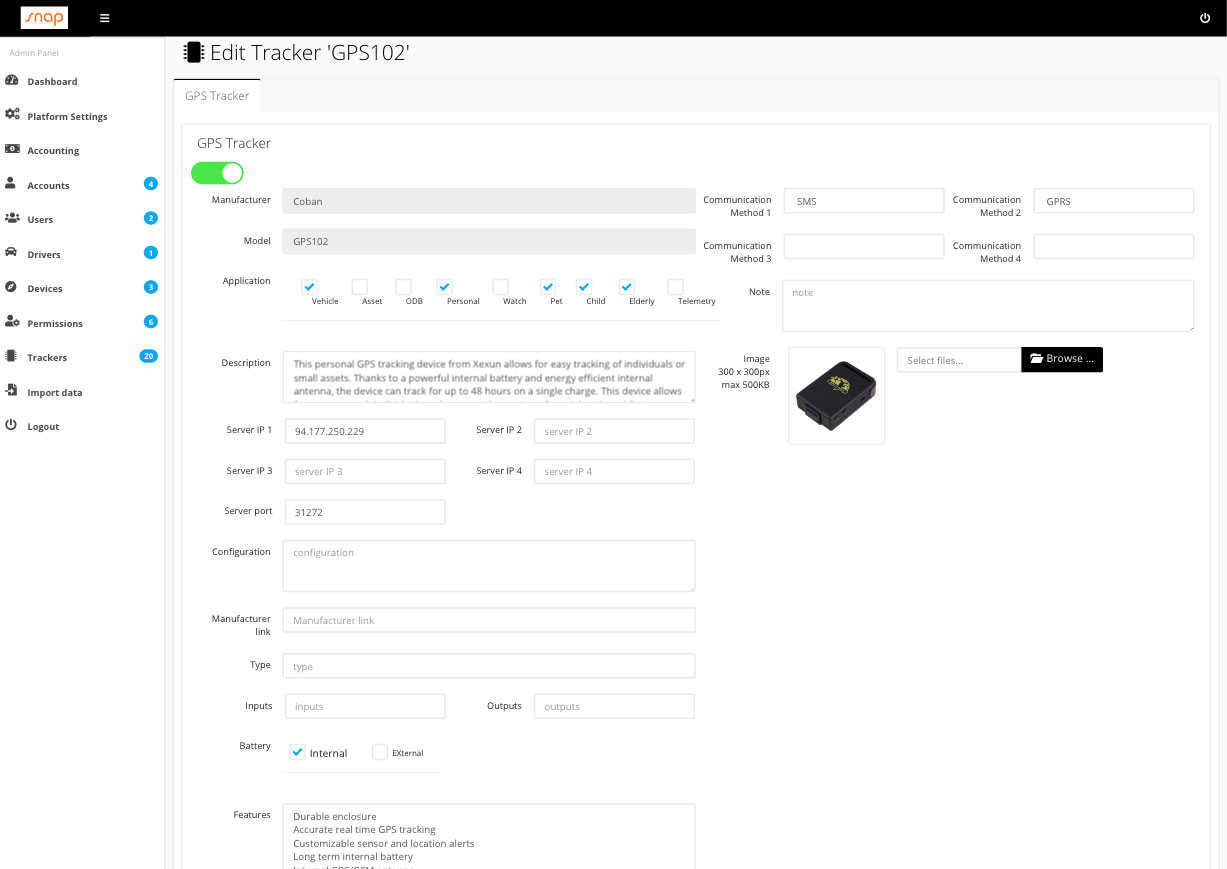The image is divided into two primary sections. On the left-hand side, there is a section that includes a black banner stretching horizontally across the top left corner. Within this banner, there is a white rectangle featuring the text "SNAP". Following this, three white lines are displayed along with a power off symbol positioned on the far right of the banner.

Below the banner, the background transitions to a light gray color, creating a segmented view. The first noticeable text in dark gray reads "Admin Panel". Under this, a header labeled "Dashboard" appears, followed by various categories: 
- Platform Settings
- Accountant Accounts

Below these categories, several items are listed with icons on the right side in light blue circles displaying corresponding numbers. These include:
- Accounts: 4
- Users: 2
- Drivers: 1
- Devices: 3
- Permissions: 6
- Trackers: 20

At the bottom of this section, there is an "Important Logout" option.

The right-hand side of the image is dominated by black color with detailed device information. It prominently features the text "ANY TRACKER GPS 102" under which "GPS Tracker" is repeated. This text is enclosed in a green oval, with the right end of the oval being white. Below, detailed specifications are provided, stating the manufacturer as "Coping" and model as "GPS 102". The application usage is diversified and includes:
- Vehicle (checked off)
- Personal (checked off)
- Pet (checked off)
- Child (checked off)
- Family (checked off)

The communication methods are listed as SMS and GPRS. Additional features include:
- Durable enclosure
- Accurate real-time GPS tracking
- Customizable sensor and location alerts
- Long-lasting internal battery

Finally, at the bottom, technical information is displayed:
- Server IP: 94.177.250.229
- Several Point: 31.272